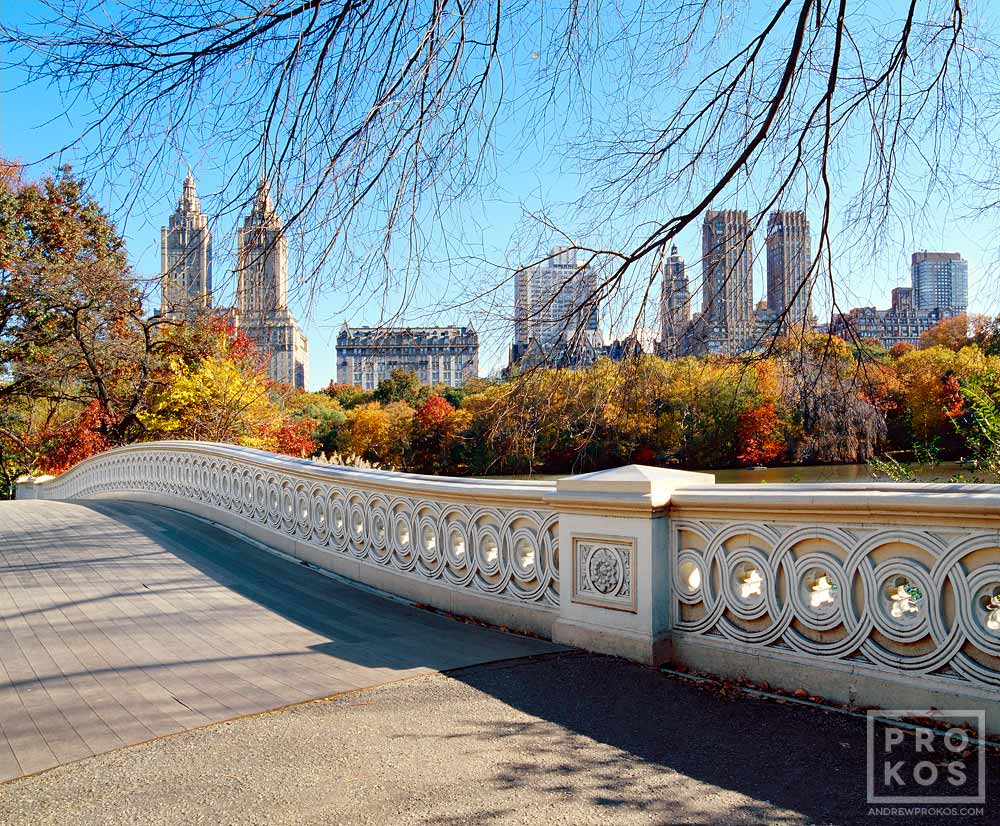This photograph captures a vibrant autumn scene in a city, possibly New York or Paris. A picturesque bridge with a stone-paved road and wooden pedestrian path spans a serene lake or river. The bridge features an elegant white stone design with interlocking circles and a cream-colored stripe along the top railing. Surrounding the waterway, a stunning array of trees displays rich fall colors ranging from reds and yellows to greens. In the background, there's a skyline featuring several tall skyscrapers, with two prominent towers on the left, followed by shorter buildings and additional high-rises. The image, taken by Andrew Prokos, is marked with his signature at the bottom right.